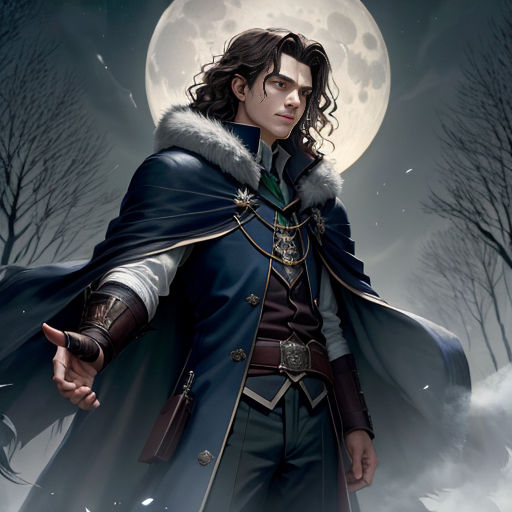In this highly detailed digital artwork, likely a CGI or cartoon-style poster, we see a serious-looking man standing against a hauntingly beautiful, moonlit backdrop. The man, with long, wavy dark brown hair, is garbed in an elaborate old-fashioned ensemble featuring a dark navy blue leather overcoat and matching trousers. His overcoat, adorned with a luxurious white fur trim around the hood, billows slightly as if caught in the wind. He wears leather wrist braces and a burgundy-brown belt that secures a sheath with a dagger on his right hip.

His refined face, marked by a strong jaw and thick eyebrows, exudes a stern and focused expression. He stands mid-thigh in the frame, extending one arm to the right with his palm open and thumb up, as if waiting for something or someone. Behind him, a massive full moon illuminates the scene, casting an ethereal glow. Dead trees frame the sides of the image, their barren branches etched against the moonlit sky filled with faint stars, creating an eerie yet mesmerizing atmosphere.